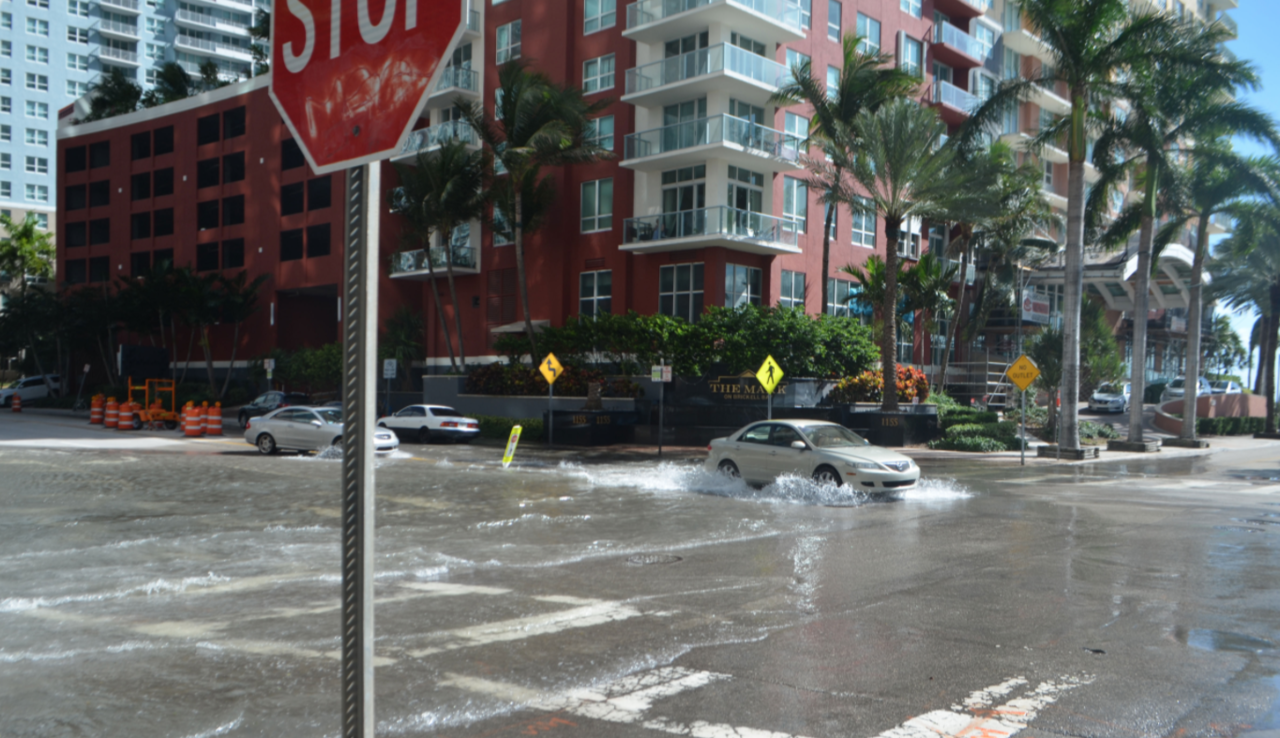This vibrant color photograph captures a daytime scene at a flooded city intersection. The sky is a clear blue, indicating a sunny day. Two cars, a silver sedan and a white sedan, are navigating through deep water, creating waves as they drive. The stop sign in the foreground adds a sense of urgency to the scene. To the right, there’s a red brick apartment building named "The Mark," featuring glass-railed balconies on the corners and an array of palm trees adorning the sidewalk in front. Traffic cones and street signs, including one marking "no outlet" and another indicating a crossing, hint at recent construction activity, possibly due to a water main break. In the background, beyond "The Mark," a taller blue apartment building adds to the urban landscape.